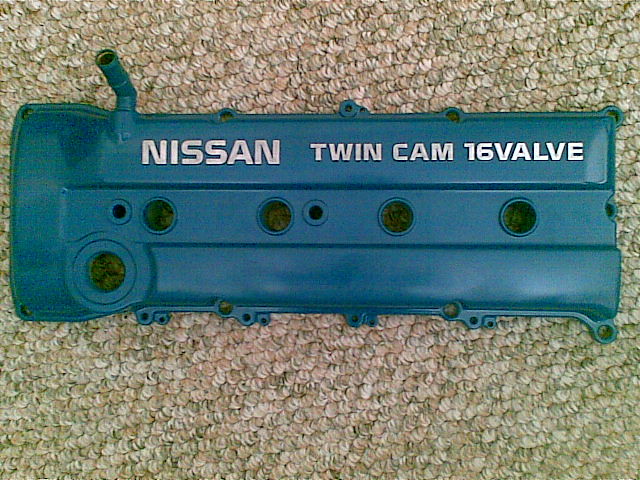The indoor color photograph features a horizontal, turquoise blue engine cover of a Nissan with the words "Nissan Twin Cam 16 Valve" in prominent white, all-capital letters across the top. The engine cover, visibly used and possibly listed for sale, is positioned on a light brown, low-pile carpet with white flecks. Central to the cover are four equal-sized circular openings aligned horizontally. In addition, there is a larger round opening located in the lower left corner and an intake valve tube protruding from the upper left corner. The entire perimeter of the valve cover is lined with holes likely meant for securing it to the engine. The cleaned and visually intact cover suggests a recent paint job, enhancing its appearance for potential buyers.